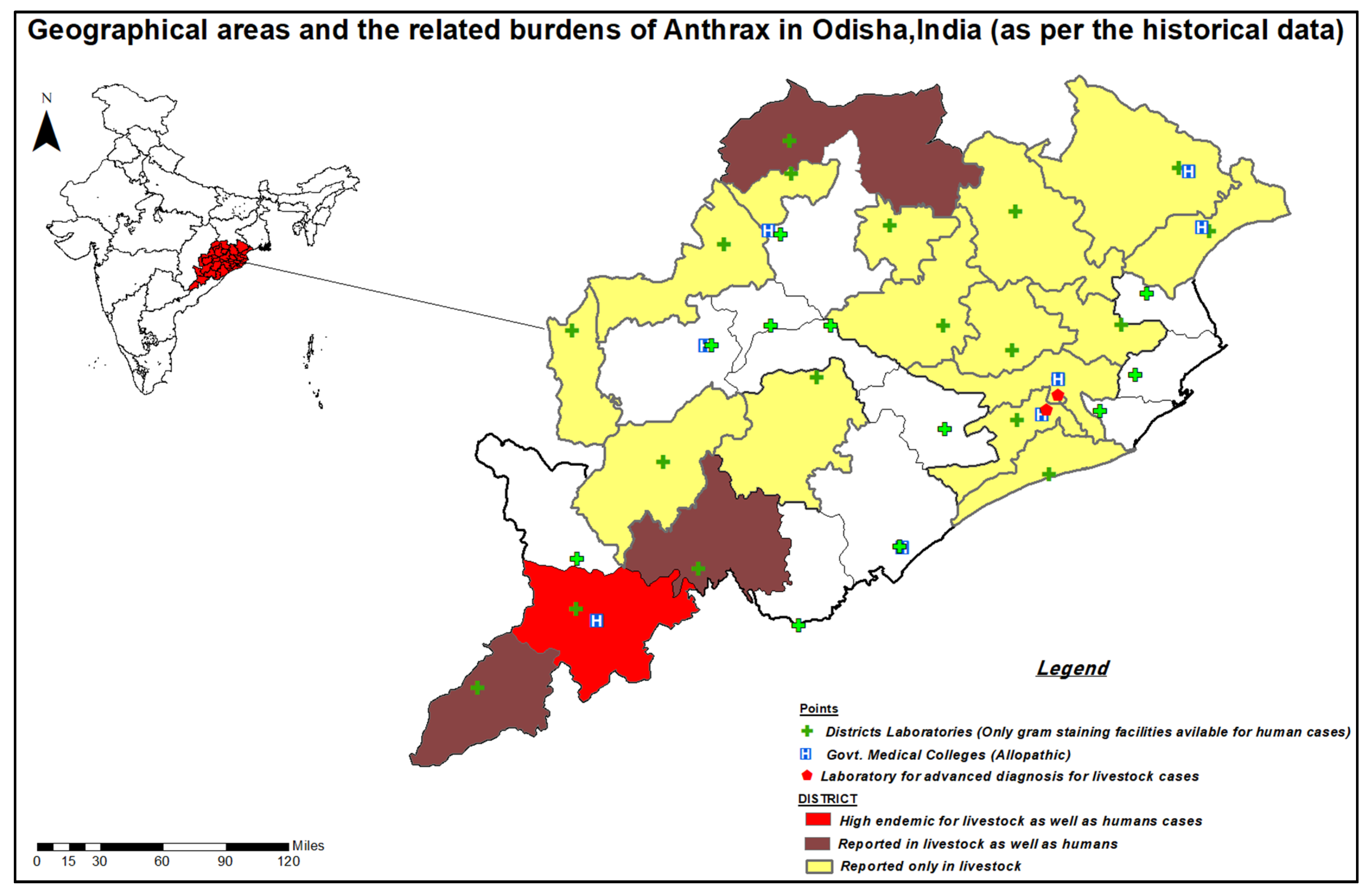"This image depicts a detailed map highlighting anthrax-related data in Odisha, India. At the top, the title reads 'Geographical Areas and the Related Burdens of Anthrax in Odisha, India as per Historical Data.' The upper left corner features a general map of India with a red-highlighted region pointing to a larger, zoomed-in map of Odisha on the right. This zoomed-in map is color-coded: red areas indicate high endemic zones for both livestock and human cases, brown areas show where anthrax has been reported in both livestock and humans, yellow areas indicate reports solely in livestock, and white areas denote no reports. The legend at the bottom clarifies that green plus symbols mark district laboratories, blue squares with a white 'H' represent government medical colleges, and red hexagons denote laboratories equipped for advanced diagnostics of livestock cases."